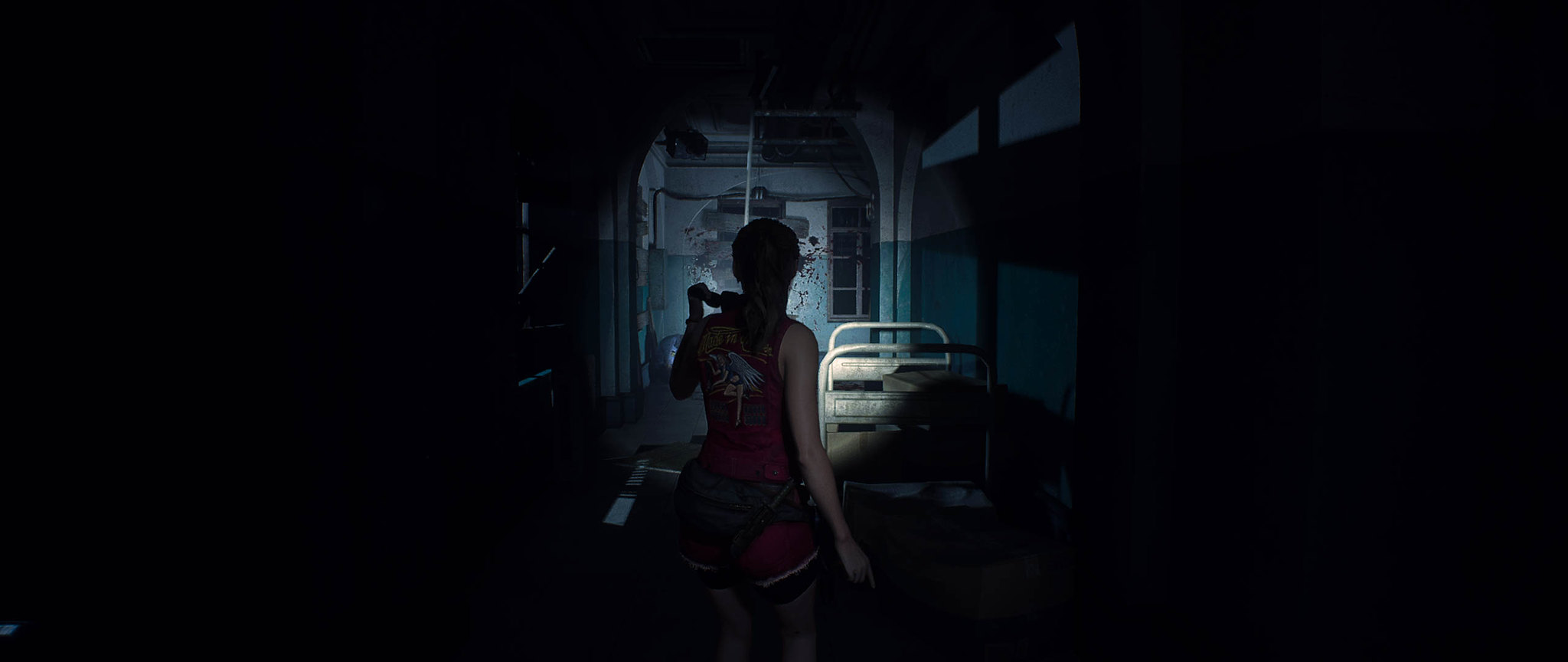In this image, we observe a video game design screen dominated by an extremely dark atmosphere, necessitating the use of a flashlight by the character featured. The majority of the image is enveloped in blackness, specifically on both the left and right sides, with the focus concentrated in the illuminated center.

The character, viewed from behind, is dressed in a purple shirt and purple shorts, complemented by a black attachment around her waist. Her right arm hangs down by her side with her index finger pointed toward the ground, while her left hand firmly grips a flashlight, casting light into the dark room.

The center of the room is dimly lit, revealing a gray object and walls with a blue hue at the bottom transitioning to gray at the top. To the right side at the back of the room, the outline of a window can be faintly seen. This detailed depiction highlights the ominous and suspenseful setting within the game, emphasizing the character's cautious exploration with the flashlight.